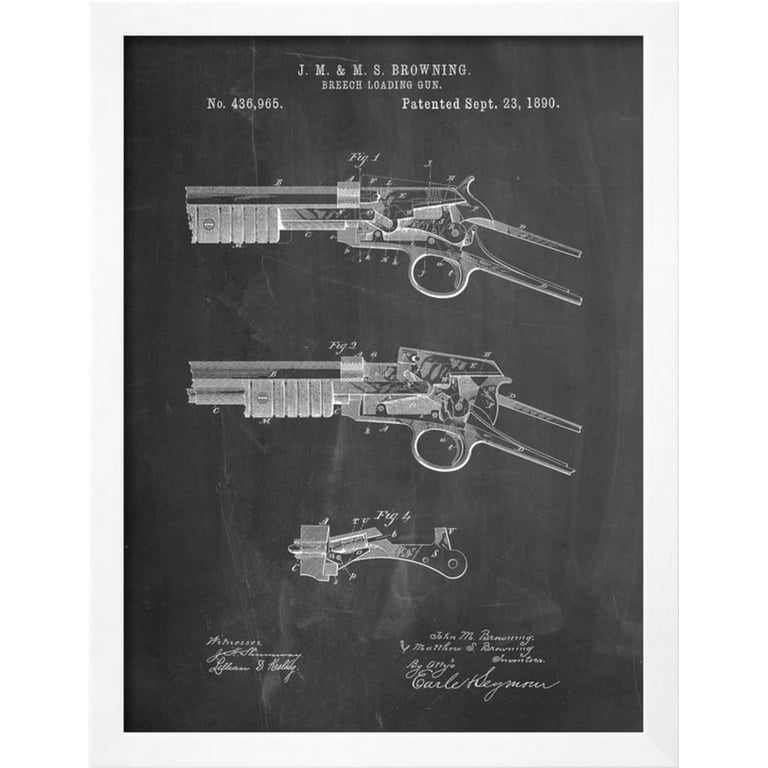This black-and-white diagram, likely resembling a patent blueprint, depicts the internal mechanisms of a J.M. and M.S. Browning breech-loading gun, patent number 436965, dated September 23, 1890. The diagram is set against a black background with white text and illustrations. At the top, it prominently displays "J.M. and M.S. Browning Breech-Loading Gun No. 436965 Patented September 23, 1890." The main illustration consists of three figures. Figure 1 provides a side profile cross-section of the gun, showcasing its internal components above the trigger and behind the barrel. Figure 2 illustrates the same cross-section but demonstrates the movement of the mechanism when the metal lever at the back is lifted. Figure 3 appears to zoom in on the handle or a smaller component of the gun. Both the left and right bottom corners of the diagram feature thin-lined signatures, including names that are difficult to decipher but may read "Matthew Browning" and "Earl Heyman" among others. The detailed renderings offer a comprehensive examination of the firearm's design and operation.